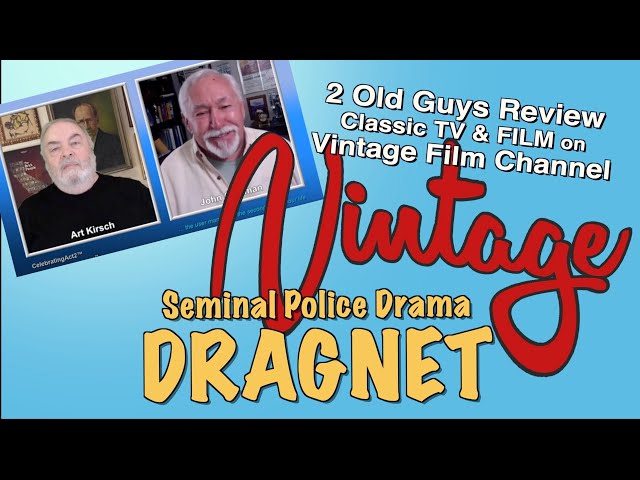The image resembles a vintage movie poster design with distinct black bands at the top and bottom, simulating a film frame. The central background is predominantly blue, and in the upper left corner, there are photos of two elderly gentlemen. One is labeled "Art Kirsch," identifiable by his black shirt, while the other remains unlabeled. Both men appear to be in their 60s, characterized by white beards and either white or gray hair. The main header in white text reads, "Two old guys review classic TV and film on Vintage Film Channel." Beneath this, in a large, stylized red script, is the word "Vintage," followed by the title of this week's episode in medium-sized yellow print: "Seminole Police Drama, Dragnet." This appears to be an advertisement for a podcast or YouTube channel where the duo reviews old movies and TV shows.